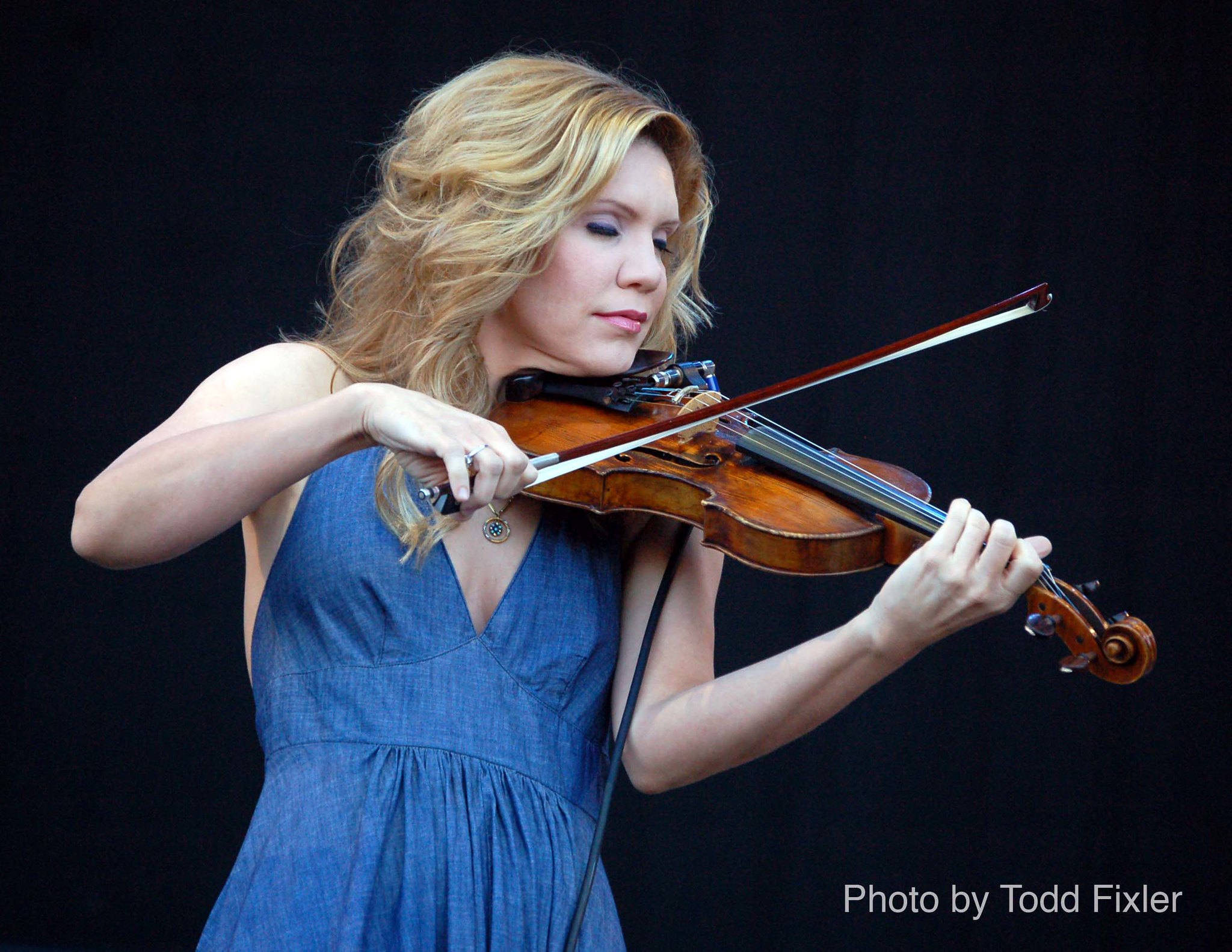In this striking image set against a black backdrop, a woman with long, slightly brown-tinged blonde hair passionately plays an electric violin. She is dressed in a sleeveless blue denim or halter dress and adorned with a necklace. Her eyes are closed in deep concentration, accentuating her pink lipstick and elaborate makeup as she immerses herself in the performance. The violin’s wooden elements are evident as she holds the strings with one hand and maneuvers the bow with the other. A black cord connected to the instrument hints at its electric nature. The overall scene, dominated by shades of black and blue, is further enriched by a watermark in the lower right corner reading "photo by Todd Fixler," indicating the photographer's credit.